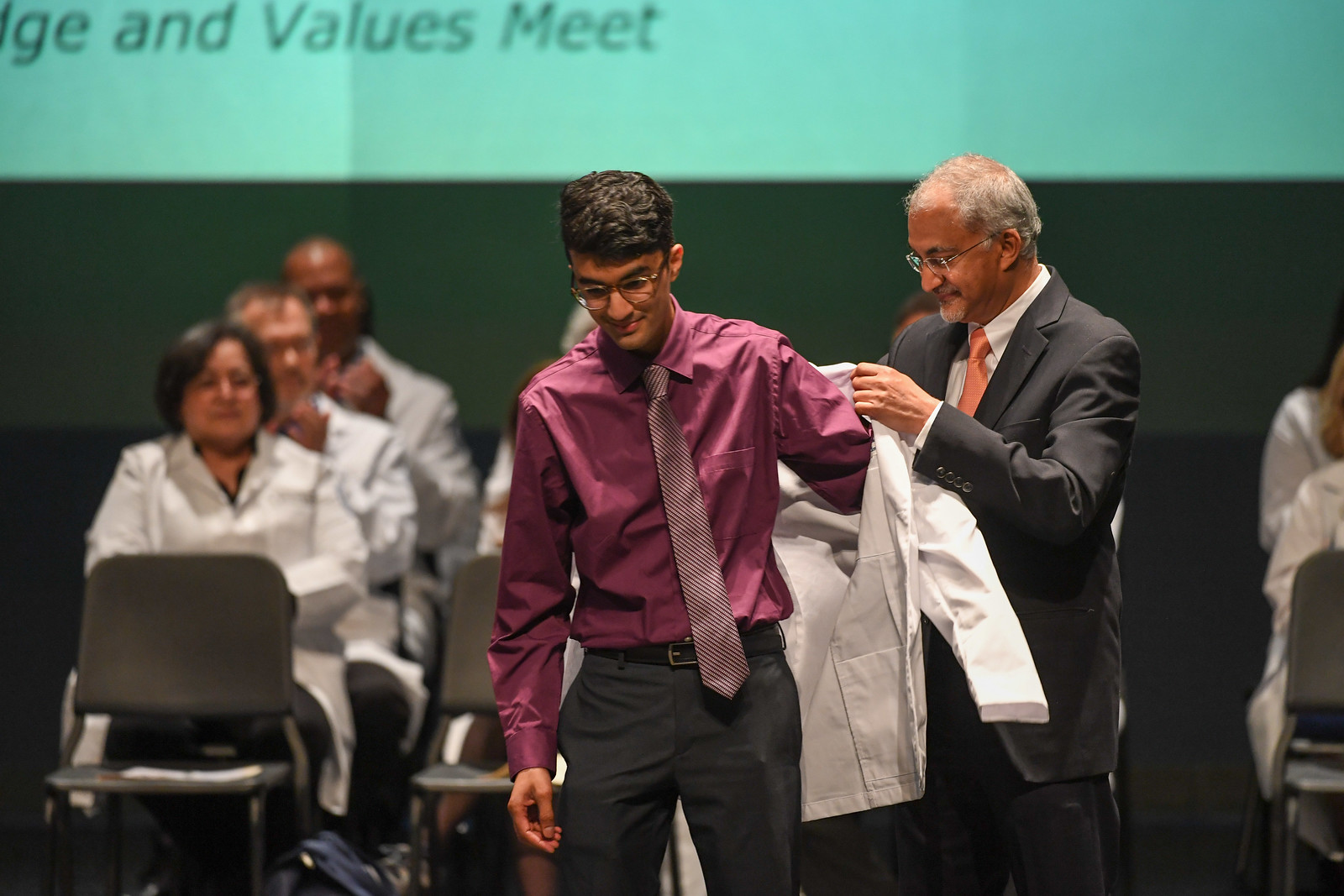In this detailed image, an older gentleman and a young man are centered in the foreground. The older man, dressed in a sharp black suit with a white shirt, an orange tie, and glasses, holds out a white lab coat for the young man. The young man, freshly shaved and clean-cut, has dark hair, glasses, and wears a maroon button-down shirt paired with gray pants and a maroon-striped tie. The older man appears to be assisting the young man in donning the lab coat, suggesting some form of ceremonial activity, possibly a graduation or a professional induction.

In the background, which features a turquoise wall with a strip of green and a darker gray section below it, there's partially visible text that reads "**and values meet**." This text is somewhat blurred and hard to read clearly. Seated in rows behind the pair are several individuals also in white lab coats, seemingly applauding, contributing to a celebratory or formal environment. Notably, there are two or three vacant seats in the front row, adding a sense of space and arrangement to the scene. The atmosphere conveys a moment of significance, likely where professional achievement and mentorship are being celebrated.